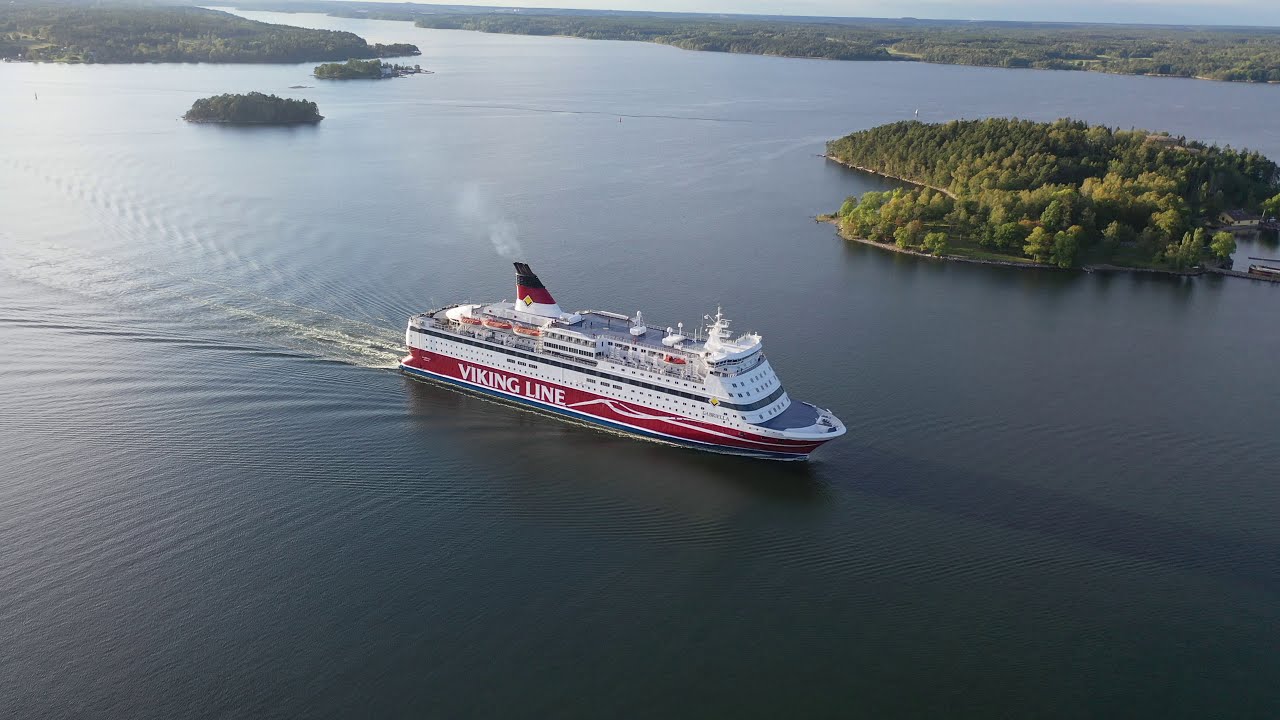The image captures an aerial view of a Viking Line cruise ship navigating through a calm and expansive body of water. The ship, prominently positioned near the center of the photo, features a white hull with a distinctive red stripe along the bottom, adorned with the words "Viking Line" in white. Above the red stripe, we see multiple decks, but no visible passengers. Puffs of smoke are seen emitting from the ship's smokestack, which is striped in white, red, and black.

Surrounding the cruise liner are several small, low-lying islands, each dotted with green trees and bushes, contributing to a scenic and tranquil atmosphere. Toward the top of the image, the water meets a broader landmass layered with greenery, while a thin, straight strip of sky is visible above the flat shoreline.

The setting suggests a mid-day outdoor scene, possibly in Scandinavia, given the Viking Line's origins and the characteristic landscape. The colors within the image include various shades of blue from the water, green from the vegetation, and the brown, white, red, yellow, and tan hues of the ship and surrounding nature. The overall tranquility and composition of the landscape evoke a peaceful cruising experience in northern climes.